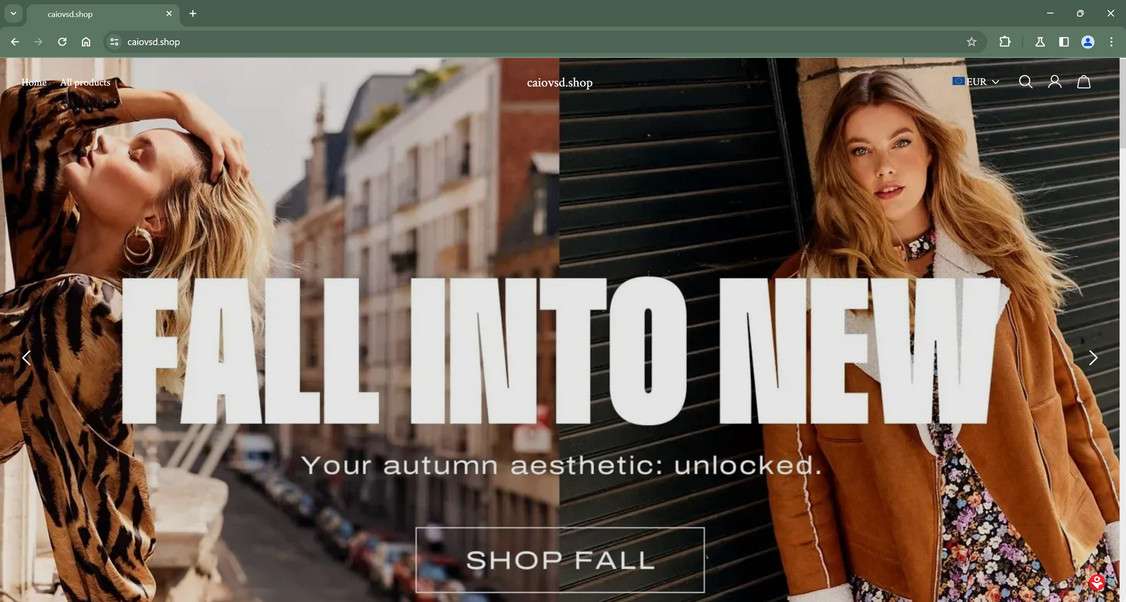Screenshot of a website displayed in a browser with a dark olive green colored navigation bar at the top, indicating only one tab open to the URL caiovsd.shop. The main webpage showcases a panoramic, landscape-style banner featuring side-by-side images of two women, capturing a vibrant autumn aesthetic. On the left, a woman with flowing blonde hair and an upward-turned gaze runs her hand through her locks. She is adorned in a tan-striped shirt and earrings, set against a backdrop of European-style buildings lining a city street with parked cars. On the right, another woman with wavy blonde hair and lipstick, her mouth slightly ajar, is dressed in a brown coat with white cuffs over a black floral-printed dress. She stands in front of black-doored, closed storefronts. Above the images, text reads "Fall into new - your autumn aesthetic unlocked. Shop fall," inviting visitors to explore seasonal offerings.